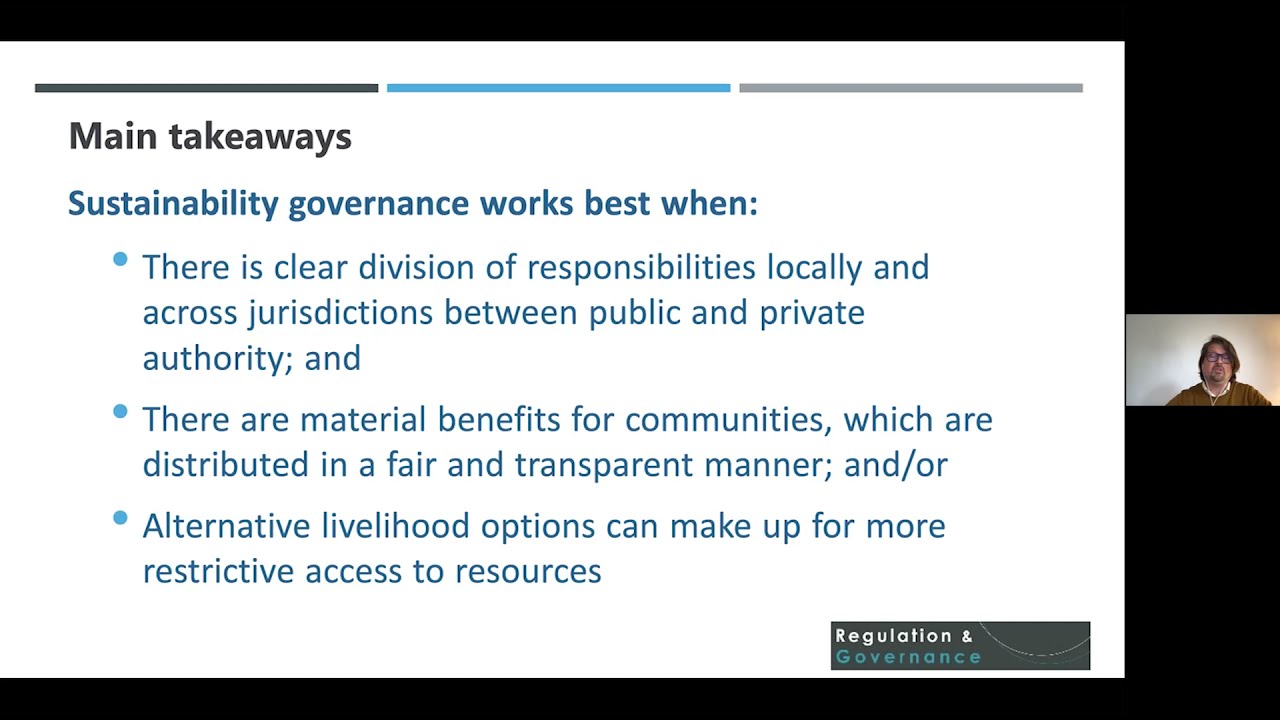The image appears to be a PowerPoint presentation slide heavily filled with text, occupying almost the entirety of the layout. The central text area is predominantly white-on-black, with several bullet points under the heading "Main Takeaways" in bold black text, followed by a primary blue subheading stating, "Sustainability governance works best when." The detailed bullet points elaborate on this theme:

- There is a clear division of responsibilities locally and across jurisdictions between public and private authority.
- There are material benefits for communities, which are distributed in a fair and transparent manner.
- Alternative livelihood options can make up for more restrictive access to resources.

At the bottom right corner of the text area in a small gray section, it states "Regulation and governance."

To the right center of the image, a small inset features a man appearing to teach or present, as if on a webcam. He wears glasses and a mustard-brown sweater over a white collared shirt, and has longish hair. The man's presence adds a personal touch to the informative and structured format of the slide. The overall color scheme of the slide includes black, white, gray, blue, and brown, aligning with common visual styles used in educational or professional presentations.